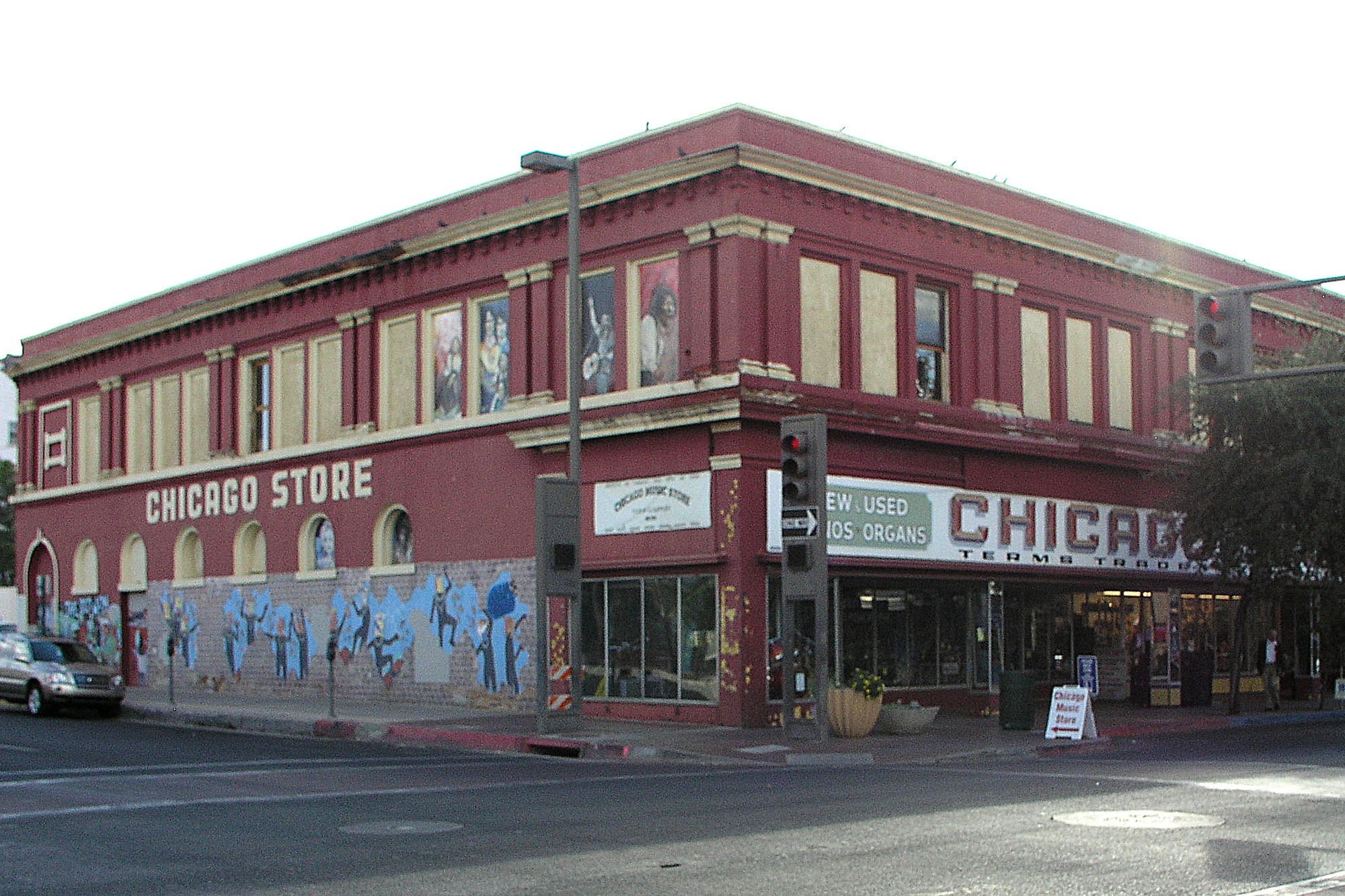The photograph captures a vibrant, large, cranberry red-brick building on the corner of a street. The storefront prominently displays "Chicago Store" in bold white block letters just below the second floor on the left side, and a large white banner above the entrance reads "New Used Organs" in striking red text. The building stands out with its detailed design features, including goldish-beige trimmed window frames, some of which have murals of artists, with one depicted holding a guitar. The lower portion of the building is adorned with blue graffiti art, illustrating people dancing in dynamic poses. The bright red and white signage is complemented by wicker baskets full of plants outside the store entrance. The scene is set against a backdrop of a gray asphalt street with a red pedestrian crossing, lined with parked cars and flanked by green trees on the right. Two streetlights, currently showing red, highlight the intersection, reinforcing the urban setting beneath a cloud-filled, bright sky that bathes the scene in diffused sunlight.